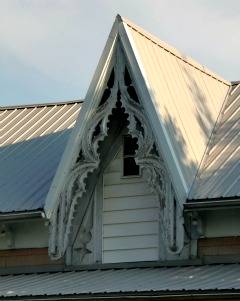This close-up photo captures the intricate detail of a dormer window on a house with a light gray metal roof. The dormer features a very small window, almost doll-sized, set against the white siding of the house. Above the window, the gable forms a sharp triangle and is adorned with elaborate, possibly carved or wrought iron artwork. There is a secondary metal ledge just below the window, emphasizing the dormer's connection to the roof. The photograph also shows how the roof seamlessly integrates around the dormer, accentuating the design with a curved pattern on either side of the gable. The background reveals a partly cloudy sky with some sun dappling on the roof, casting shadows of branches. This image highlights a tiny yet complex architectural segment.